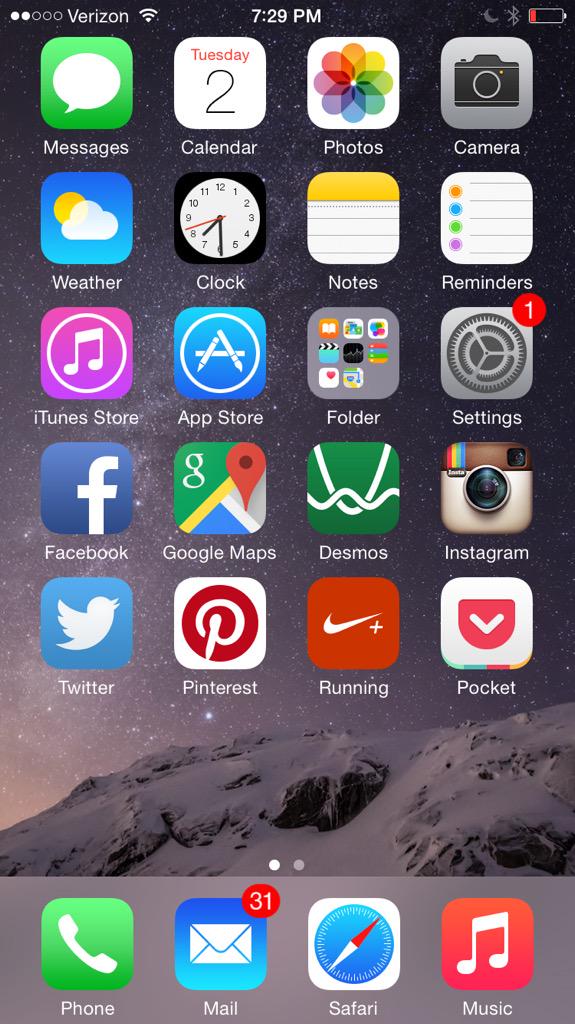The screen capture depicts the app screen of an iPhone, showcasing an organized array of applications against a stunning background. The wallpaper features a serene night sky filled with twinkling stars, overlaying a majestic snow-covered mountain at the bottom. 

At the top of the screen, the status bar indicates the iPhone is connected to the Verizon network, with the current time displayed as 7:29 PM. The battery icon, showing just one red bar, suggests that the phone is in urgent need of charging.

The main app screen is arranged in a grid of five rows, each containing four apps. The first row includes essential applications such as Messages and Calendar, while subsequent rows feature popular apps like Facebook, Google Maps, and Instagram. The final row includes Twitter, Pinterest, the Nike Running Club app indicated by the Nike logo, and Pocket.

At the bottom of the screen, the dock retains the four default iPhone apps for quick access: the green Phone app, the blue Mail app, the blue Safari browser, and the red Music app. This layout offers a blend of utility and accessibility, common in standard iPhone configuration.